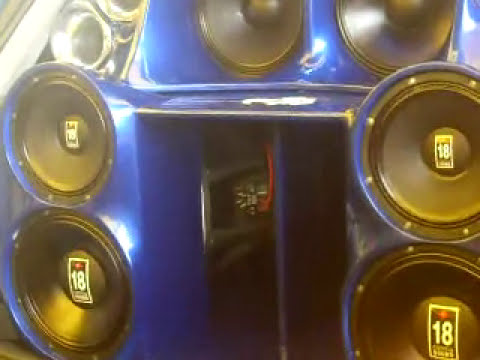The photograph depicts a set of high-powered speakers encased in blue enameled boxes, marked with the number "18" on their labels in white text. The image features three sets of speakers: two standing upright on either side and one lying flat on top. These speakers, possibly woofers, display metallic round objects and are primarily black in color with silver trimming. A red cord is plugged into the middle speaker, suggesting a powered setup. The photograph, which is four inches by four inches, is of medium to low quality with artificial lighting, suggesting an indoor setting. The blue coloration predominantly features in the encasements, with the circular black speakers prominently standing out. While initially appearing automotive, they could also form part of a larger speaker stack or amplifier system.